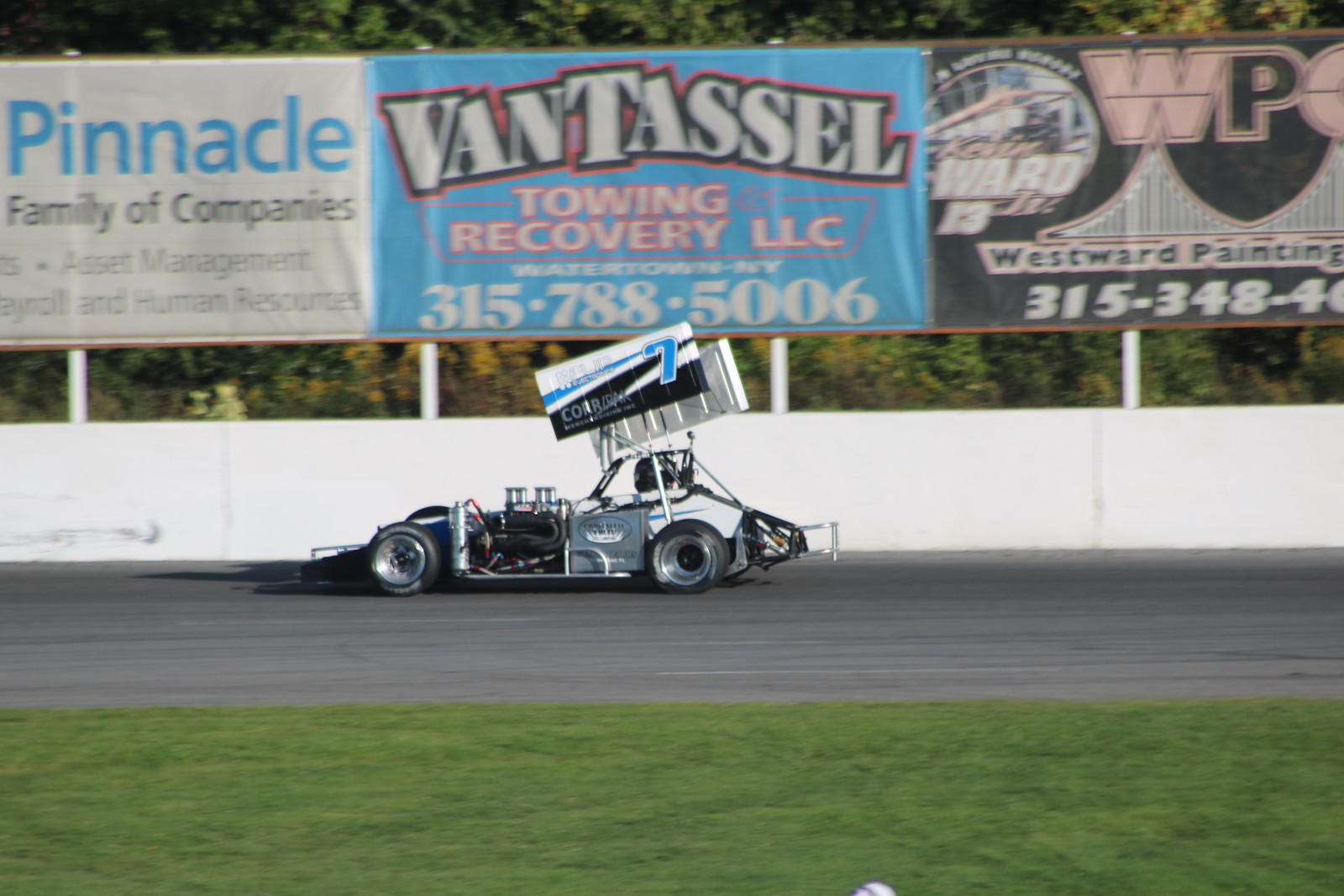The photograph captures an outdoor racetrack scene during the daytime, showcasing a unique race car resting on the asphalt, which spans horizontally across the middle of the image. The car, slightly left-of-center and oriented towards the left side of the frame, is predominantly white and gray with its front engine mostly exposed due to the hood being removed. A large wing is positioned atop the driver's seat area, giving the car an unconventional appearance. Prominently featured on the car is a black, white, and blue poster displaying the number 7 in blue. Surrounding the racetrack is a white wall intended to protect bystanders, adorned with three sponsor banners, namely Pinnacle, Van Tassel, and Westward Painting, which offer contact information. These banners are mounted on white posts, contrasting against the backdrop of dense woods. The foreground is accentuated by a stretch of green grass, enhancing the vivid realism and photographic representationalism of the scene.